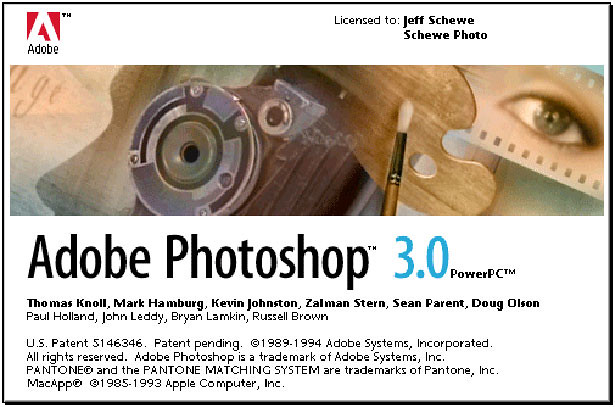The image features a splash screen for Adobe Photoshop 3.0, set against a white background with a black border. In the top left corner, the Adobe logo is prominently displayed with the word "Adobe" beneath it. On the top right, the text reads, "Licensed to Jeff Schewe, Schewe Photo." Central to the image is a horizontal photo illustrating a composite of elements, including a woman's eye, a painter's palette with brushes, and a section resembling the front of a camera. Below this, the heading "Adobe Photoshop 3.0" stands out, with "3.0" in blue text, followed by "PowerPC™" and a list of names and credits in black text. The credits include notable contributors such as Thomas Noll, Mark Hamburg, Kevin Johnston, Zalman Stern, and others. Additional information includes a U.S. patent number, trademark notices, and a copyright statement from 1989-1994 by Adobe Systems Incorporated. This nostalgic splash screen encapsulates the early branding and interface of Adobe Photoshop.